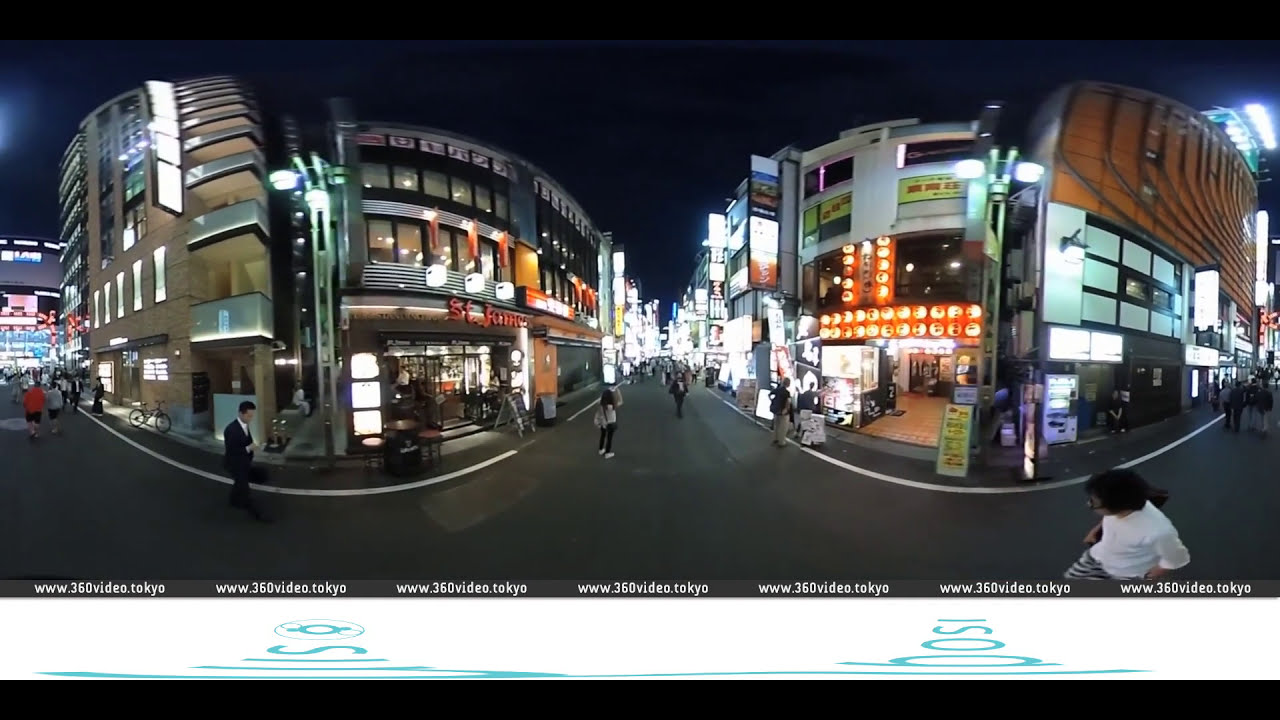The image is a dynamic and bustling nighttime street scene in downtown Tokyo, captured through a fisheye lens that distorts and rounds the edges, giving it a panoramic feel. The sky is a deep navy blue, almost black, indicating the late hour. The street is brimming with pedestrian activity, with no cars in sight, suggesting it's a dedicated pedestrian pathway flanked by shops and modern buildings lit up brightly. Large business fronts line both sides, some towering three to four stories high, adorned with a multitude of vibrant advertisements and neon signs. The colors in the scene range from black, white, gray, and silver to more vibrant hues like red, orange, yellow, pink, and brown. A businessman, clad in a suit, is engrossed in his phone amidst a crowd of people engaged in shopping, taking photos, and exploring the area. Distinct paper lanterns, colored in orange and lit up in yellow, hang on one of the buildings, further adding to the ambiance. At the bottom of the image, a watermark repeatedly states "www.360video.tokyo," emphasizing its origin and the likelihood that it’s part of a live streaming setup from a website.